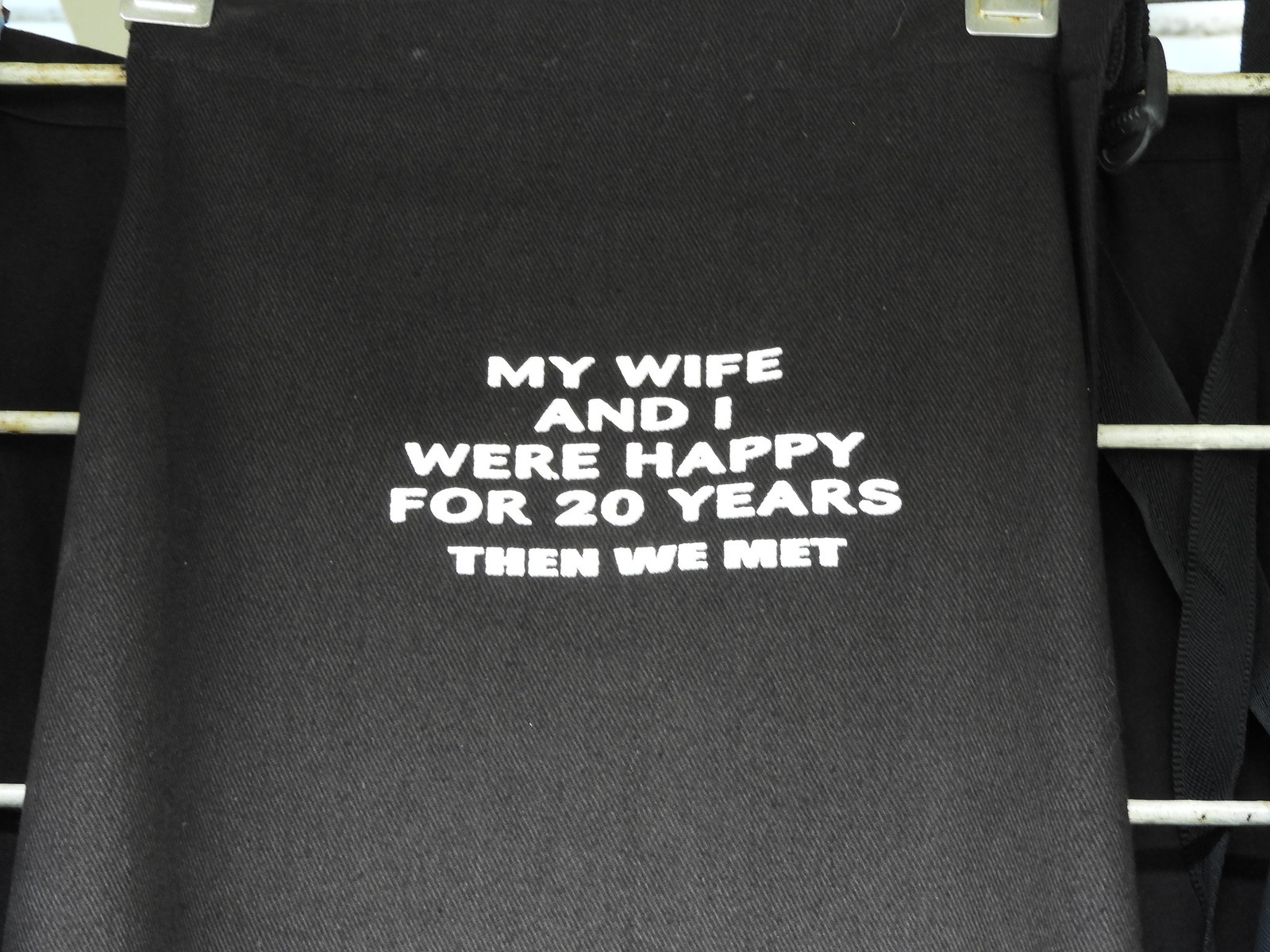The image features a black piece of fabric, likely a shirt, towel, or bag, prominently displayed and held in place by two silver clips at the top, which are partially visible. The fabric is draped over three horizontal white rods, possibly a drying rack, that extend from left to right across the frame. In the center of the black fabric, written in white text, are the words: "My wife and I were happy for 20 years, then we met." The background consists primarily of black, with another piece of black fabric and a black strap visible. The photograph appears to be taken from above, looking down at the setup.